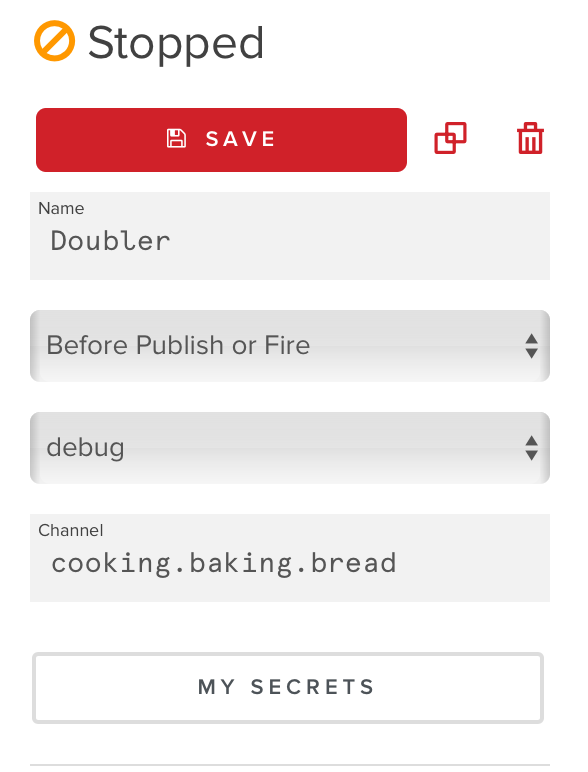The screenshot appears to be from a mobile application with a minimalist design featuring a solid white background with light gray sections for different input fields. At the top, bold black text reads "Stopped," with an adjacent orange circle containing a line through it, likely indicating a paused or inactive status.

Directly below, a prominent red button labeled "Save" in white text is featured, accompanied by a small clipart icon of a floppy disk. To the right of this button, there are two clipart icons: one resembling a copy symbol and the other a trash can, likely for duplicating or deleting content.

Beneath this row is a gray section titled "Name," within which the word "Doubler" has been entered. The next section is also gray and indicates a drop-down menu with the current selection reading "Before, Publish, or Fire." Following this is another similar drop-down menu with "Debug" as the selected option.

Further down, another gray section labeled "Channel" contains text that reads "Cooking.Baking.Bread." At the bottom of the screen, there is a white button outlined in the same light gray found in the input sections, and it reads "MY SECRETS" in uppercase letters. A subtle light gray line runs along the very bottom of the screenshot.